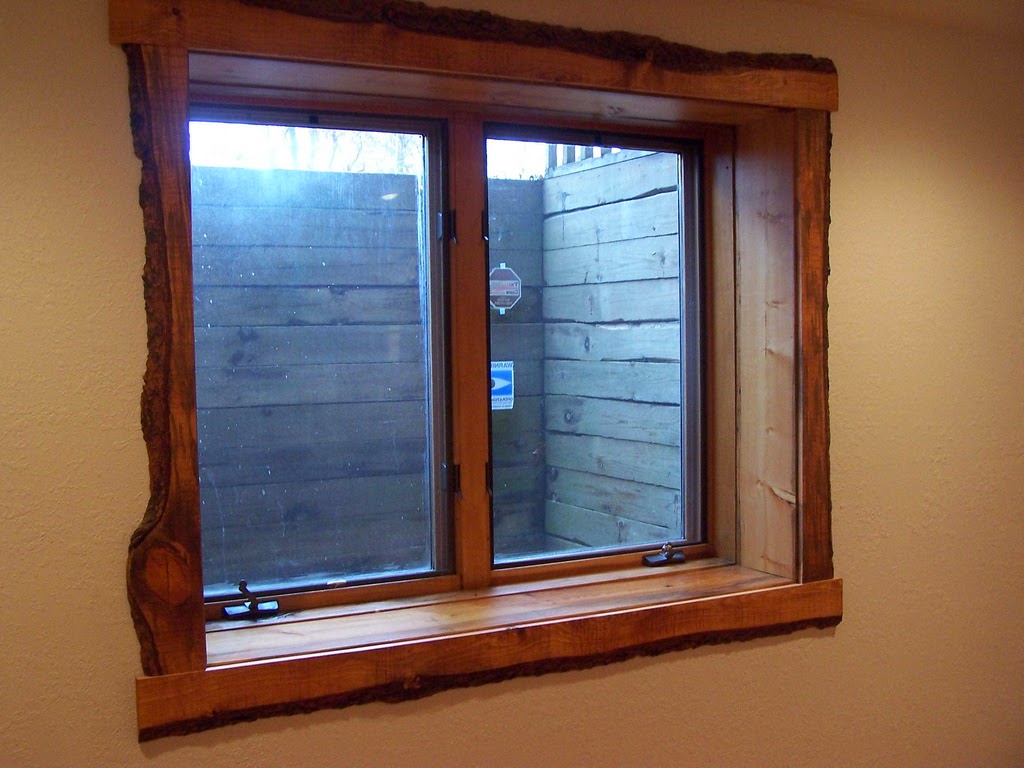This photograph captures an interior view from a window set into a light yellowish wall, possibly in a basement. The window, framed with heavy, possibly rough-finished wood resembling freshly cut logs, showcases two panes designed to slide open horizontally. Beyond the glass, a walled-off area suggests a patio or foundation, constructed from broad, rough wooden planks stacked about ten high. Sunlight filters through, illuminating trees just above the wooden barrier. Additionally, two signs with unreadable text are affixed to the wooden wall outside, with at least one displaying blue and white colors. Black latches secure the rustic dark brown wood-trimmed window, ensuring it commands the central focus of the image, while the encompassing scenery hints at a serene outdoor section of the house.